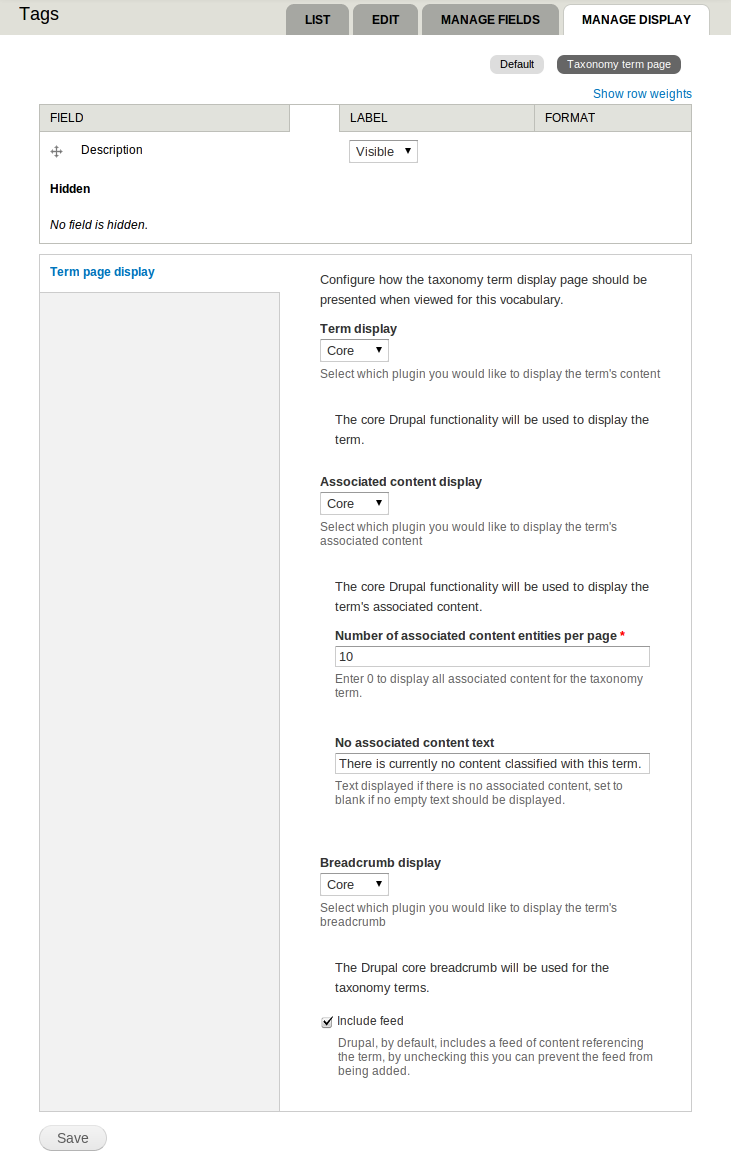**Detailed Caption for Screenshot:**

This screenshot provides an extensive guide on how to manage and display taxonomy terms within a Drupal content management system. The interface highlights various sections including "Edit Manage Fields" and "Manage Display," emphasizing the "Default" text option. Several parameters can be configured:

1. **Tagging and Selection Options** - Users can manage the fields and edit the display options for taxonomy terms.
2. **Visibility Settings** - The interface specifies whether fields should be visible or hidden; it notes that currently no field is hidden.
3. **Term Page Display** - Detailed configuration on how the taxonomy term display page should be presented is shown, with the core functionality outlined.
4. **Associated Content Display** - A core feature allows selection of plugins to display associated content for terms, reinforcing that the Drupal core functionality will be utilized for this display.
5. **Pagination and Text Options** - Set the number of associated content entities per page (default is 10), and control settings to "Enter 0 here to display all associated content." Additionally, customize the "No Associated Content" text to inform users when there is no content linked with a term.
6. **Additional Settings** - The display core can be included or excluded for feeds.

The screenshot clearly illustrates the layout and options available for efficiently managing taxonomy terms and associated content within Drupal.